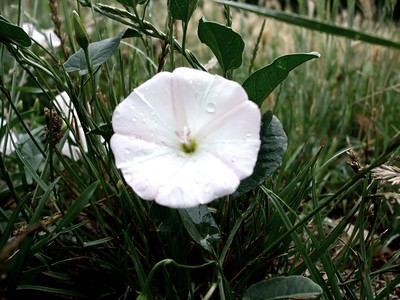This close-up image captures a beautiful white morning glory flower in full bloom, situated outdoors amidst a natural setting. The flower's round, large petals exhibit a delicate, barely-there pink shading that subtly enhances its pristine white color. At the center of the flower, a greenish hue highlights the entirety, accentuating the delicate stamens that emerge from the core. Tiny droplets of dew cling to the petals, adding a touch of morning freshness to the scene.

Around the base of the flower, dark green leaves intertwine with various shades of grass, from deep green to lighter tones, extending into the background. The grass appears taller and sparser as it recedes, transitioning to patches of light tan and brown, suggesting a dry or transitioning season. On the left side of the image, there are blurry hints of additional flowers, though they remain out of focus and secondary to the central bloom. The bottom right corner reveals a glimpse of brown vegetation and partially visible soil, grounding the lush greenery in an earthy context.